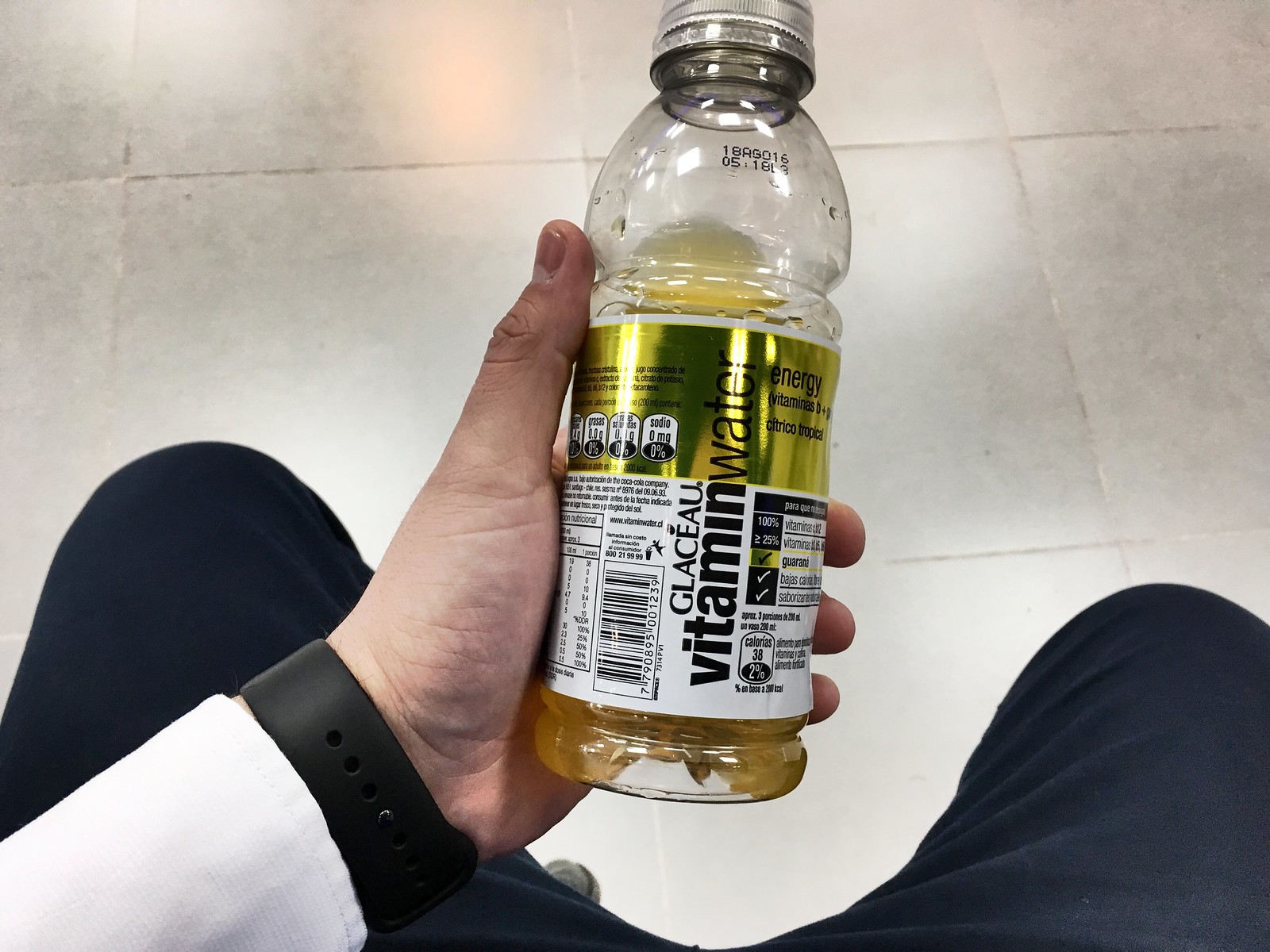In this top-down photograph, a person's perspective captures their left hand holding a clear plastic bottle of yellow, tropical-flavored Vitamin Water. The bottle features a gold label at the top, transitioning to white with nutritional information towards the bottom, and it is capped with a silver lid. The individual, seated possibly on a stool, wears black jeans, a white long-sleeved shirt, and a black wristwatch on their left wrist. The setting is a glossy, white tile floor with large tiles, which extends beyond the edges of the image. The bottle is positioned centrally in front of the person, with about half of its contents remaining. The scene also shows the tip of the person's toe peeking into the frame at the bottom.